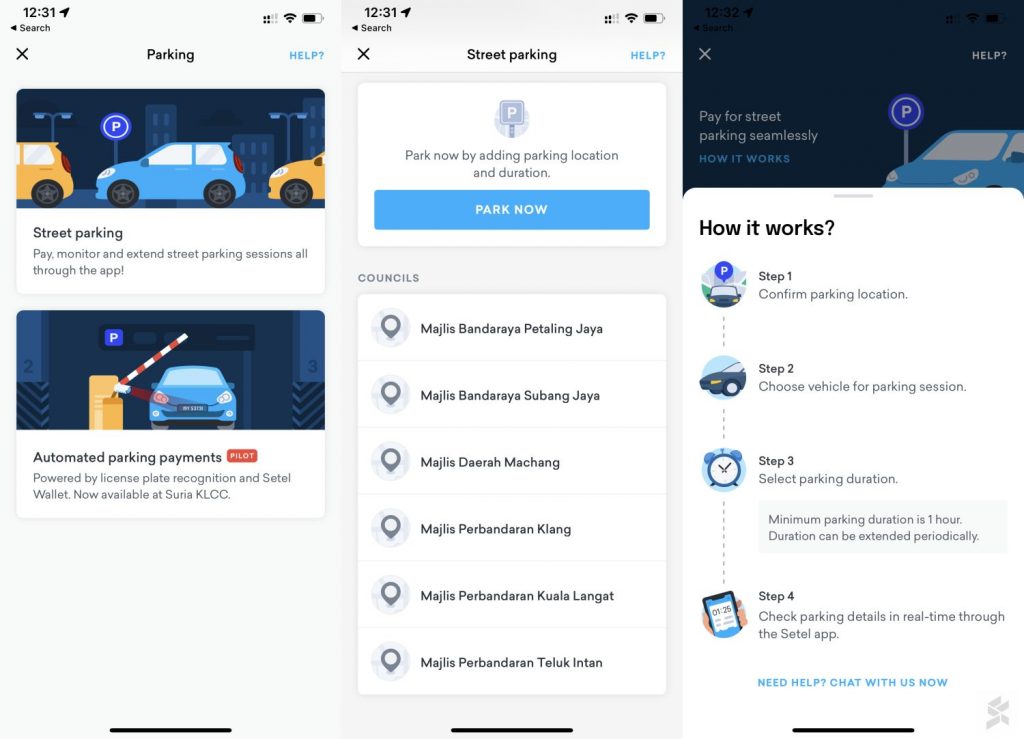### Detailed Caption for the Image Series

The image consists of three vertically aligned screenshots from a parking app. Here's a detailed description of each segment from left to right:

**Left Image:**
- **Header:** The top bar displays the time as 12:31, along with icons for Wi-Fi, battery charge, and signal strength.
- **Search Bar:** Just below the time, there is a search bar with a "Search" input field and a button next to it.
- **Title and Help:** The main section is titled "Parking" and includes a clickable green question mark icon with the word "Help" to the right.
- **Top Illustration:** Features a cartoon illustration of a blue car parked parallel between two yellow cars, with a blue parking sign (a blue circle with a white "P") behind the blue car, set against a dark cityscape. This section is captioned: "Street Parking - Pay, Monitor, and Extend Street Parking Session All Through the App!"
- **Bottom Illustration:** Titled "Automated Parking Payments," this part shows a blue car facing the viewer underneath a raised red and white striped gate arm at a parking garage entrance. The gate arm is mounted on a broad yellow post, with a parking garage seen in the background. There's also a red button (text unreadable) and additional text indicating the use of "License Plate Recognition" and mentioning it's available at Surya KLCC.

**Middle Image:**
- **Header:** Similar to the left image, the top bar shows the time as 12:31, Wi-Fi, battery charge, and signal icons.
- **Title and Action Button:** Titled "Street Parking," this section features a prominent, clickable blue rectangle reading "Park Now."
- **Instructions:** Above the "Park Now" button, the text reads "Park Now by Adding Parking Location and Duration."
- **Council Options:** Below, there's a white box listing six options relating to different areas, starting with "Magis Bhandaraya Hetaling Jaya," followed by options like "Subang Jaya," each with an inverted teardrop-shaped location pin icon.

**Right Image:**
- **Header and Title:** The top black section includes an image of the same blue car in front of the blue parking sign, with text reading "Pay for Street Parking Seamlessly: How It Works."
- **Instructions:** The main white section offers a four-step guide titled "How It Works":
  1. **Confirm Parking Location:** This step is illustrated with a car icon under a peace sign.
  2. **Choose Vehicle for Parking Session:** Depicted by an icon of a car's front end.
  3. **Select Parking Duration:** Represented by an alarm clock icon. Additional box text reads "Minimum parking duration is one hour. Duration can be extended periodically."
  4. **Check Parking Details:** Illustrated by a smartphone screen in a hand, with text instructing users to check parking details in real-time through the SETEL app.

Each step in the rightmost image includes a small thumbnail illustration in a circle, corresponding to the described action.